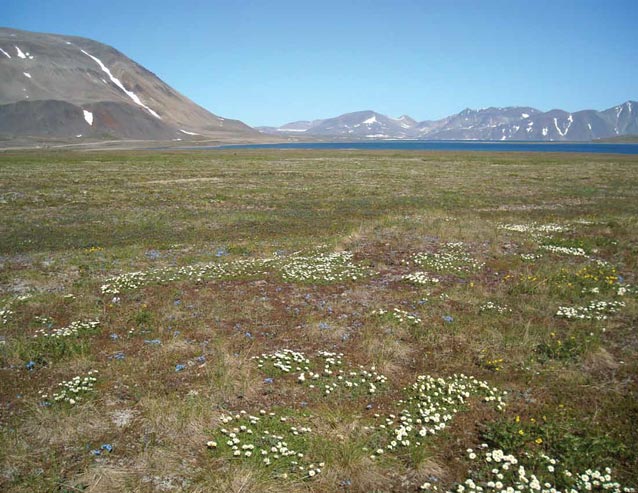The photograph captures an expansive, lightly maintained open field with a mix of patchy green and brown grass. Scattered across the ground are small wildflowers, primarily white, with occasional blue or bluish-purple ones, reminiscent of weeds. The landscape, mostly barren, features a small mound and a few patches of dead grass. In the distance, a serene, clear blue lake contrasts with the impressive backdrop of mountains and hills, some with remnants of snow that appear to be melting. The sky above is a vivid blue, cloudless and sharp, adding to the idyllic and tranquil feel of the location, ideal for a quiet outing or playing with a dog. Overall, it presents a pristine and untouched natural scene with no visible signs of human or animal activity.